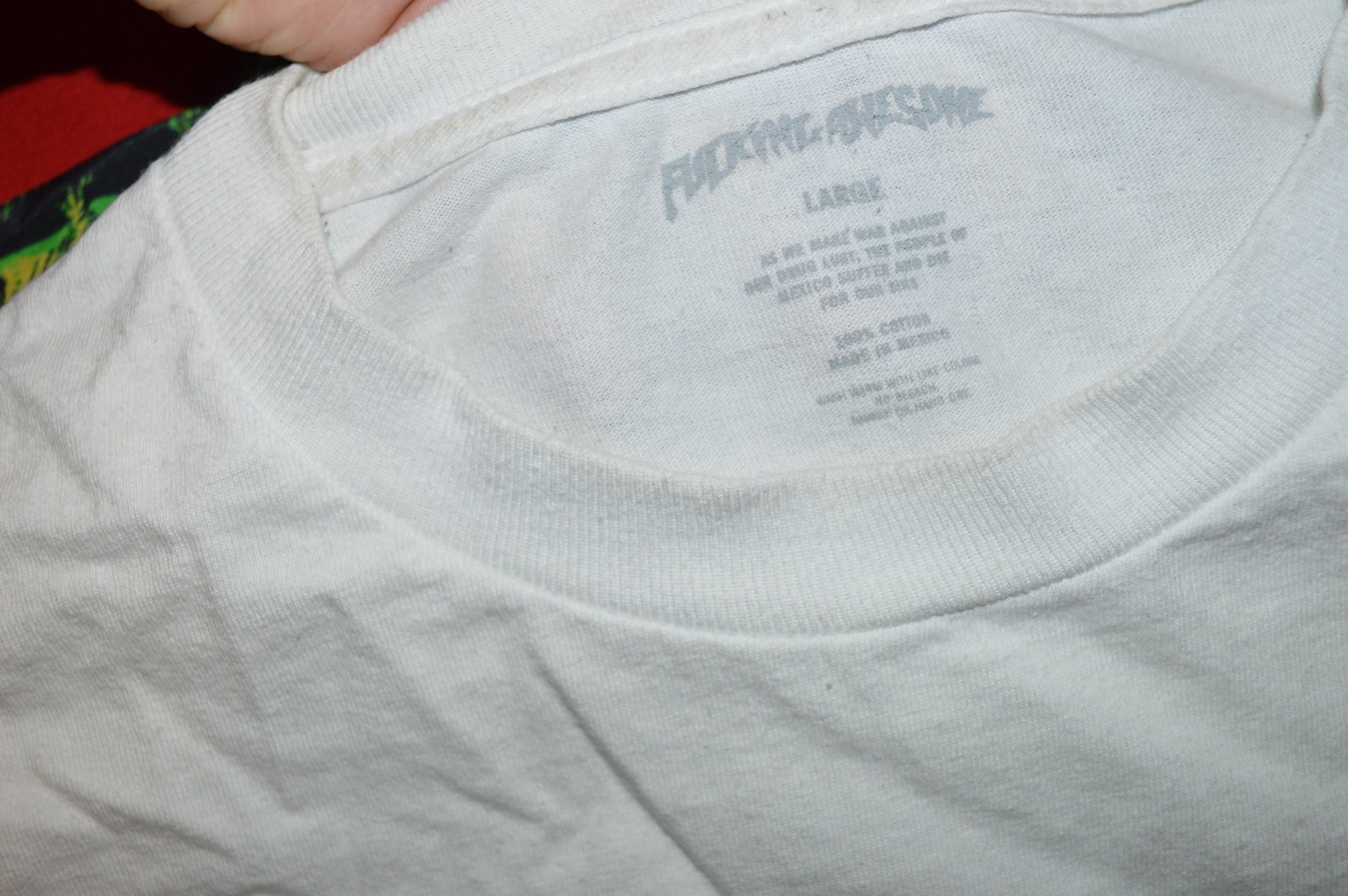This image is a close-up photograph capturing the upper portion of a wrinkled, white t-shirt, focusing mainly on the collar and the tag inside the shirt. The shirt, which takes up almost the entirety of the image, is held close under someone's chin, with a hand partly visible in the upper left corner. The label on the shirt starts with an unreadable brand name followed by the word "awesome." The tag indicates that the shirt is a large size and includes a paragraph stating, "As we make war against our drug of choice, the people of Mexico suffer and die for our sins." It also mentions that the shirt is 100% cotton and made in Mexico. Despite being mostly clean, there is slight dirt visible around the collar area. The background features indistinguishable colors in red, black, green, and yellow.